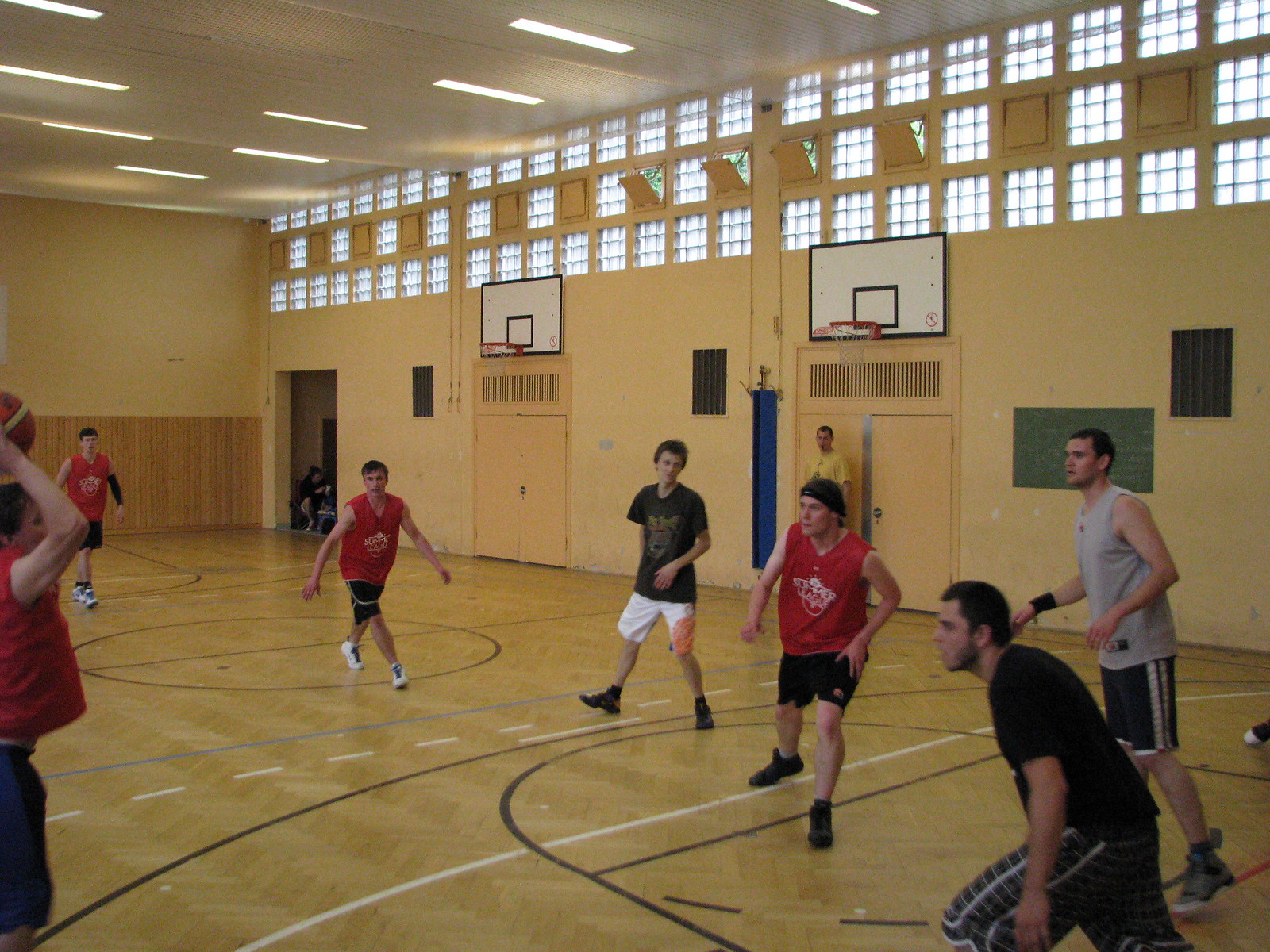This photograph captures a lively basketball game in what appears to be a high school gymnasium, characterized by its yellowish tone. Seven young men are visible on the court, all dressed in assorted athletic wear, including short-sleeve and sleeveless tops paired with shorts and sneakers. The team in red shirts and black shorts stands out, with one player prominently holding the basketball overhead on the right side of the frame, poised to pass. Positioned on the foul line is another player from the same team, ready to receive the ball, while a defender in a black shirt and white shorts closely follows him. In the paint, a taller player wearing a gray tank top and dark shorts towers over the others. On the lower left-hand side, another player in a black T-shirt focuses intently on the man with the ball. Trailing behind are two more players in red shirts, spaced roughly 10 feet apart. The back wall of the gym features two unused basketball hoops, flanked by doors, and is crowned with a strip of checkered windows near the ceiling. The gym’s recessed fluorescent lighting adds to the utilitarian aesthetic of the space.